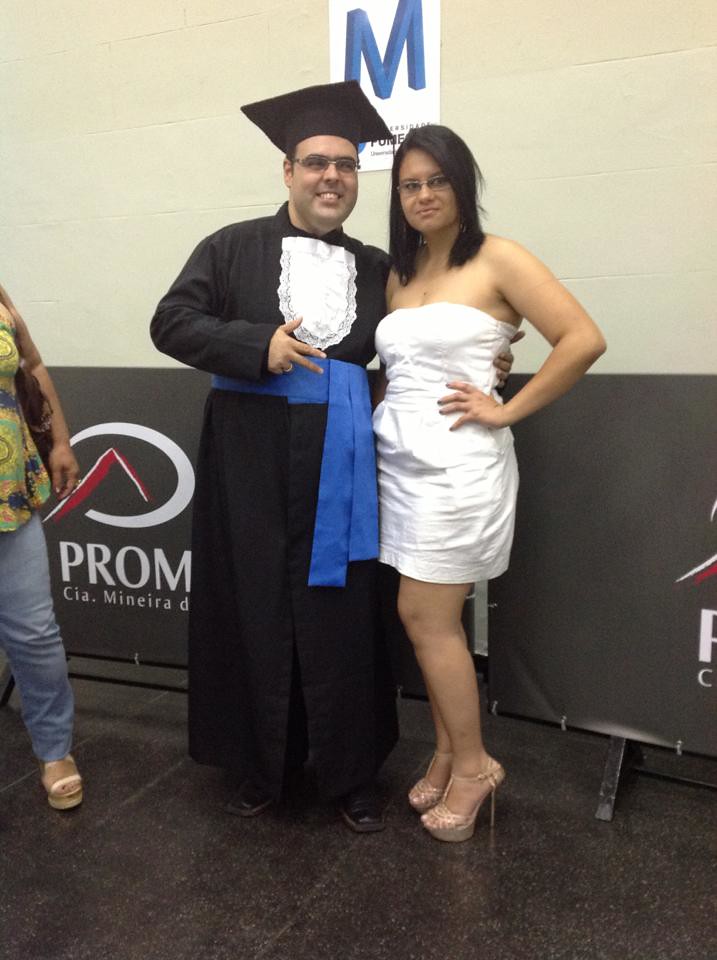The indoor photo showcases a PhD graduate and a young woman posing together. The male graduate, aged around 30 to 40 years, is dressed in traditional black graduation robes with a blue belt, and he is wearing glasses. Standing to his right, the young woman is adorned in a sleeveless, white short dress paired with beige, open-toe high heels. She also wears glasses and has black mid-length hair. The background of the image features a school gym wall decorated with a post board that reads "PROM," indicating that the event might be taking place during a graduation prom. Part of another person's body is visible in the frame, though their face is cropped out.